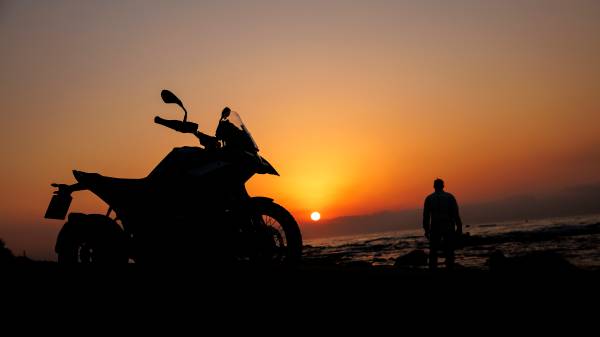This photograph, taken in an outdoor setting during late evening, captures the striking silhouette of a man standing beside a parked motorcycle on a ground area. The entire scene is enveloped in a low-quality, blurry resolution, which renders the details indistinguishable and leaves their shapes in black. The backdrop features a body of water, presumably an ocean, appearing grayish in the dim light. Highlighting the scene is the vivid sunset; the sun, positioned just above the horizon, glows white and is circled by a spectrum of colors. The sky transitions from a bright burnt orange near the sun, fading into gold, yellow, and reddish hues, eventually blending into a dark bluish tone as it extends upward. Overall, despite the image's low resolution, the magnificent colors of the sunset dominate, creating a vivid and captivating contrast against the silhouetted figures and the tranquil ocean.